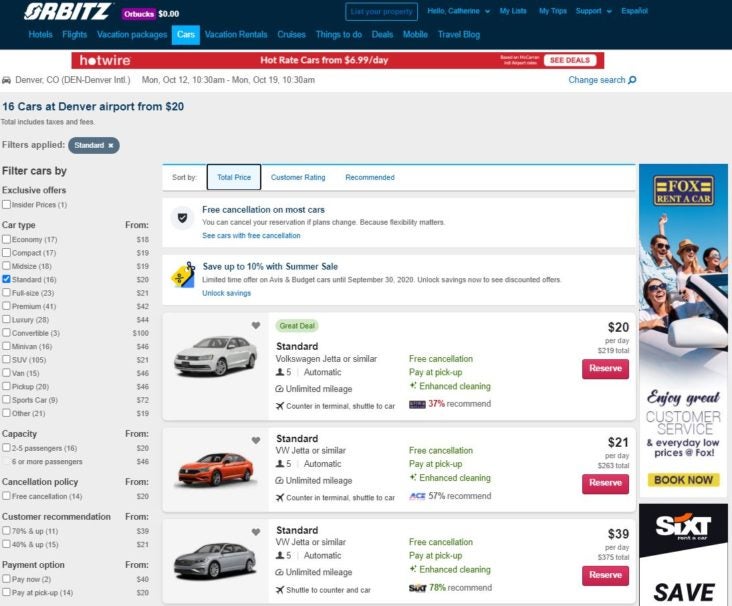On the Orbitz car rental page, the user is presented with various car options available at Denver Airport. Orbitz—an established brand in travel bookings—features an eye-catching pink-highlighted section called "Orbucks," where customers can potentially earn rewards through their rentals, though this user currently has none.

The page reveals that the user has sorted the 16 available vehicles by total price and filtered the results to show only standard vehicles, starting at a reasonable rate of $20. No other filters, such as capacity, cancellation policy, customer recommendations, or payment options, have been applied.

The results display three standard vehicles: 
1. A Volkswagen Jetta or similar, which seats five people and is priced at $20.
2. Another Volkswagen Jetta or similar, also accommodating five passengers, but priced slightly higher at $21. Despite the similar description, the car appears different in the image provided.
3. A third Volkswagen Jetta or similar option, similarly seating five people, available for $39.

The pricing differences suggest variations in features or conditions, though all vehicles fall under the same category and model specification.